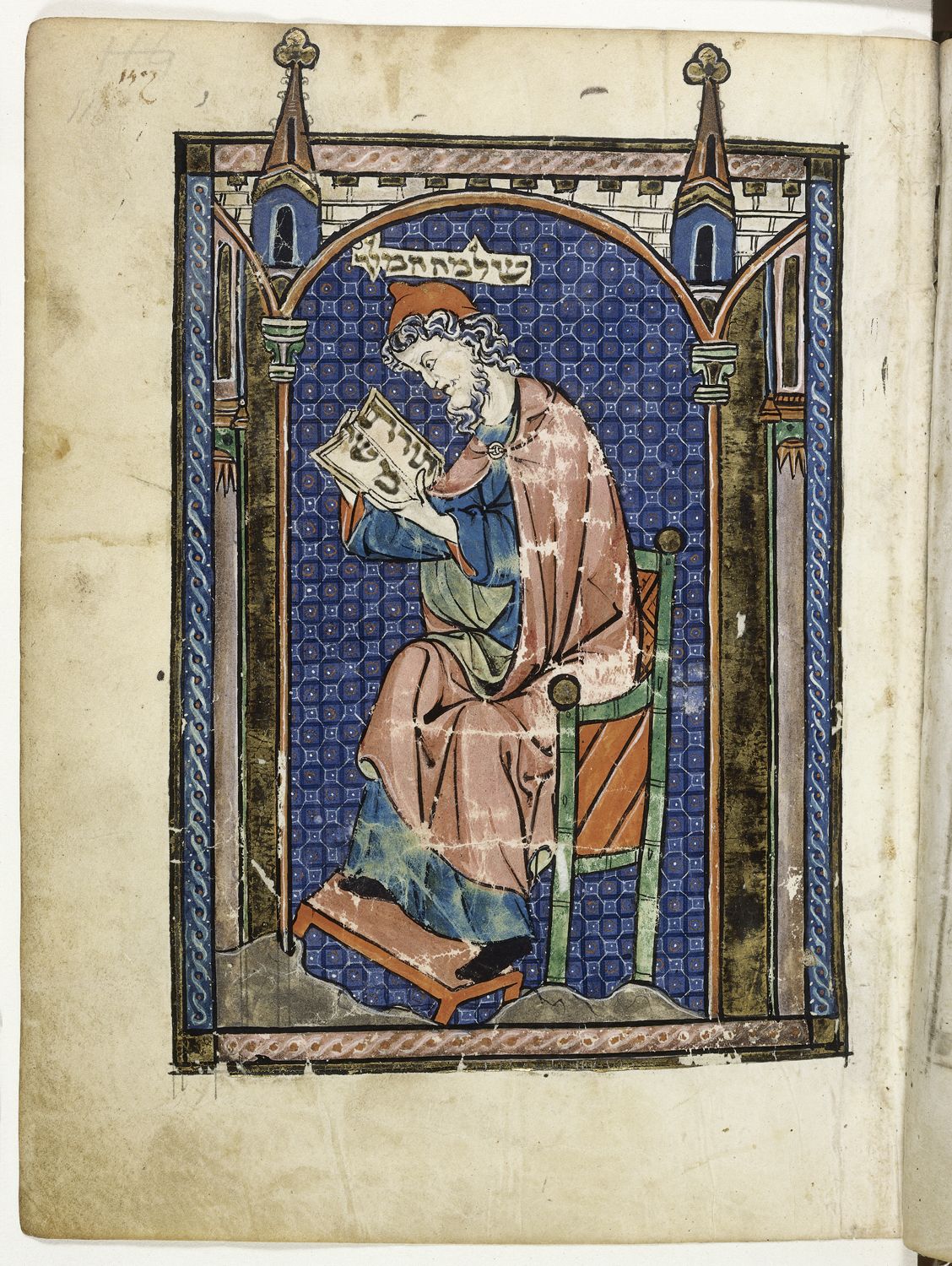This image is a rectangular painting, approximately six inches high and four inches wide. The top left and entire bottom of the image feature a light white background, juxtaposed with a weathered yellow piece of parchment that occupies the rest of the space. The parchment is marked with smudges and stains, giving it an old, antique appearance. 

The focal point of the painting is a man seated on a throne, his feet resting on a small stool as he bends over to read a paper. He has curly black hair, a beard, and wears a small brown cap. His facial expression conveys anger. Draped in a long, flowing red cloak, the man also wears a blue tunic that extends down to his feet, which are clad in black slippers. Behind him, a blue tiled wall serves as the backdrop.

The scene is encased within what appears to be parts of a scroll, with the image extending off-screen to the right. Blue downward spirals adorn the left and right sides, while two castle spires are depicted at the top. The painting might represent a stained-glass window due to its intricate and vibrant details. Despite the rich visual elements, the identity of the man and the precise narrative remain unclear.